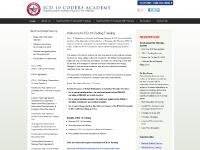Screen capture of a web page depicted with a small rendering and very fine print, making the text largely illegible and possibly not in English. At the top left of the page is a circular logo featuring a star, while to the right of this logo is some text that remains unreadable even when the resolution is increased to 200%. Below the logo is a black horizontal ribbon with white text that likely serves as navigation tabs. The main content area appears to contain a text document, flanked by sections on the left and right that possibly include additional information and references. This layout suggests that the web page might be from an official government website or a scholarly source, such as an academic institution's repository for research articles or news. However, due to the blurriness of the image and the small font size, precise identification is challenging.